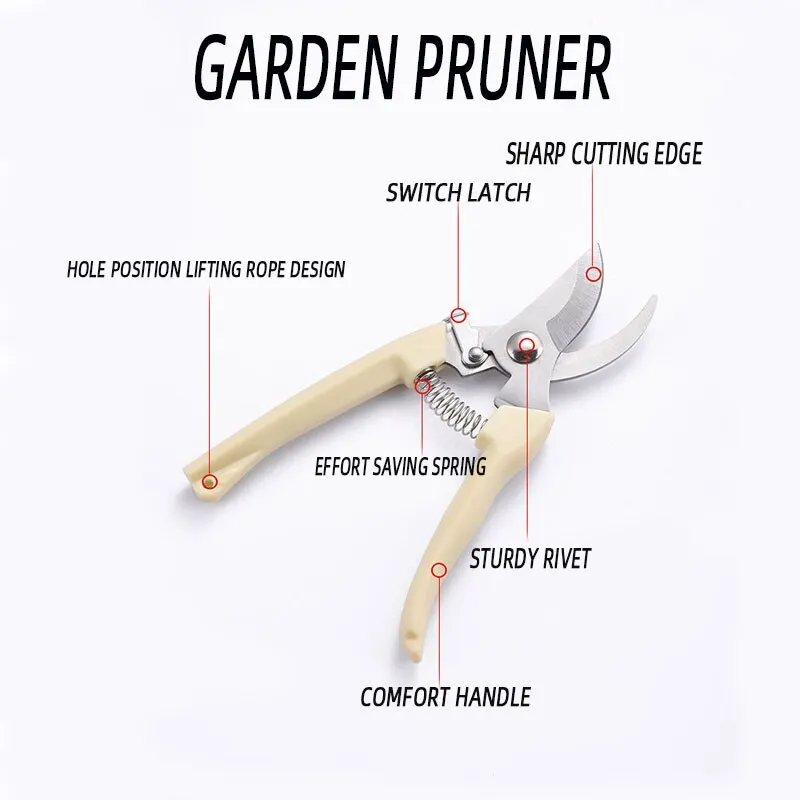This diagram illustrates a pair of garden pruners against a white background with black font labels. The pruners feature cream-colored handles and a silver cutting tool. A silver spring is positioned between the handles. At the top, the text "Garden Pruner" is displayed in black font. The central image showcases the pruners using several labeled annotations. 

At the top, near the blades, a red circle highlights the "Sharp Cutting Edge." Moving downward, another red circle marks the "Switch Latch," which is linked to a silver component of the pruners. The "Effort Saving Spring" is indicated between the handles, designed to ease the cutting action. Further down, a circle at the bottom of the handle denotes the "Whole Position Lifting Rope Design." Another red circle illustrates the "Sturdy Rivet" located just below the blades, ensuring the tool's durability. Finally, a red circle points to the "Comfort Handle," emphasizing the ergonomic design for user comfort.